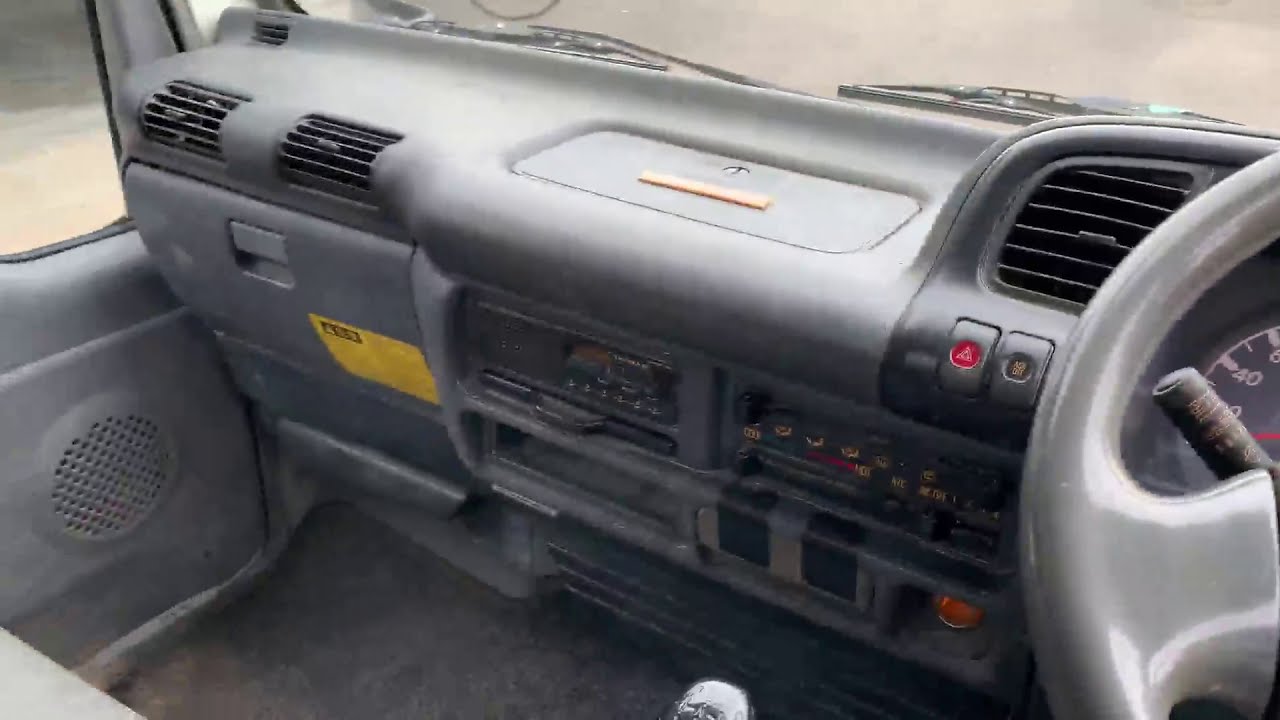This is a highly detailed, stylistic photograph depicting the interior of a vehicle, likely a car or truck, taken from the front driver's seat in landscape orientation. The interior, predominantly gray, showcases a meticulously detailed dashboard featuring various controls including those for the air conditioning and radio. The steering wheel, positioned on the right side of the image in a European style, is partially visible along with the speedometer just behind it. The dashboard also reveals several vents, a prominent white hazard button, and numerous other buttons. 

A speaker with perforated holes is embedded in the left door panel beneath a visible window. There is a flat, inset glove box on the top of the dashboard on the passenger side, distinguished by a small key lock and a yellow sticker. Another compartment on the lower dashboard front features a gray handle and an additional yellow sticker, further complemented by two vents. The floorboard, partially visible, is covered with dark brown carpet. The upper edge of the windshield reveals the windshield wipers and a long stick, which could be part of the rearview mirror assembly or another dashboard feature. The overall photographic style captures the realism and intricacies of the car’s interior.